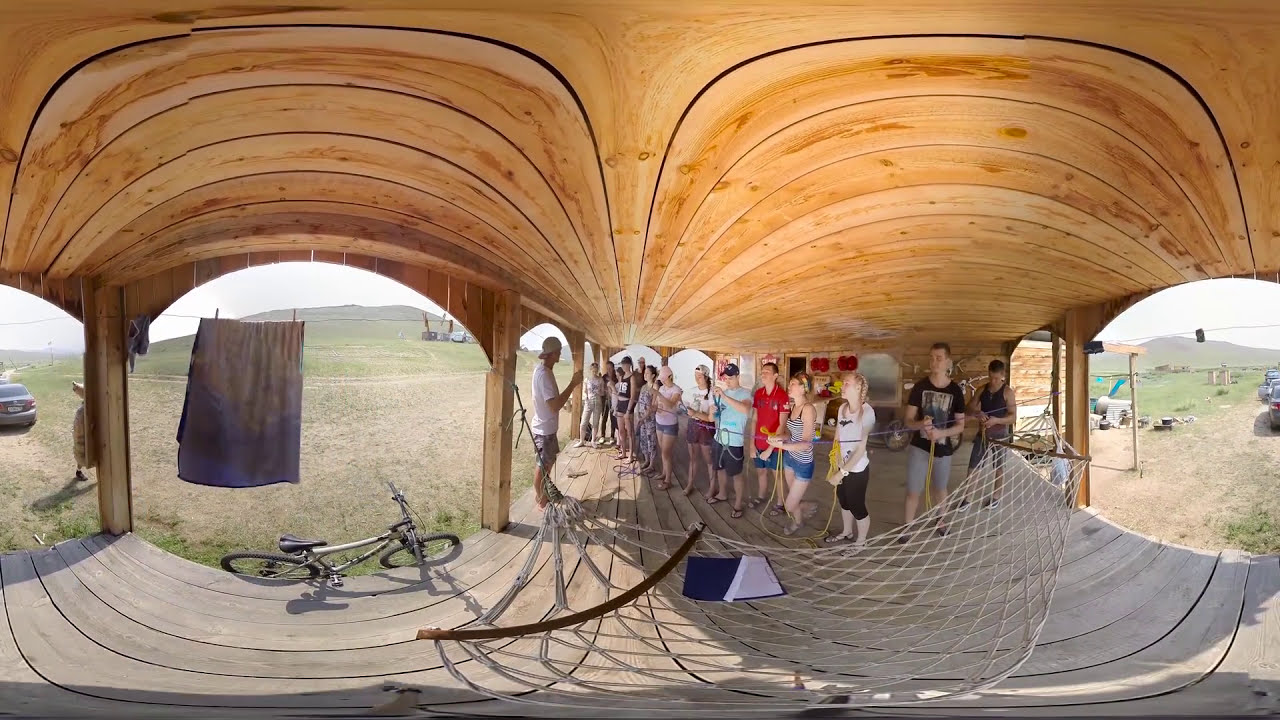In the panoramic photo, a large group of young adults, possibly teenagers on a field trip, stands in line under a uniquely built wooden structure resembling an upside-down boat with two arches stretching from the far left to the far right. A gentleman appears to be addressing them in the center of the image. The structure, made of light-colored wood with knot holes in the ceiling, features weathered, gray-colored wooden flooring. There are wooden pillars supporting the gazebo, and a beige hammock hangs from them, stretching from the center to the right. A white bike rests against the deck to the bottom left, while a dark gray car is visible on both the far left and right sides of the photo. Outside the gazebo, the scene extends into a grassy field with green and brown patches, hills in the background, and a small road in the left corner. A towel hangs on the left arch of the building.